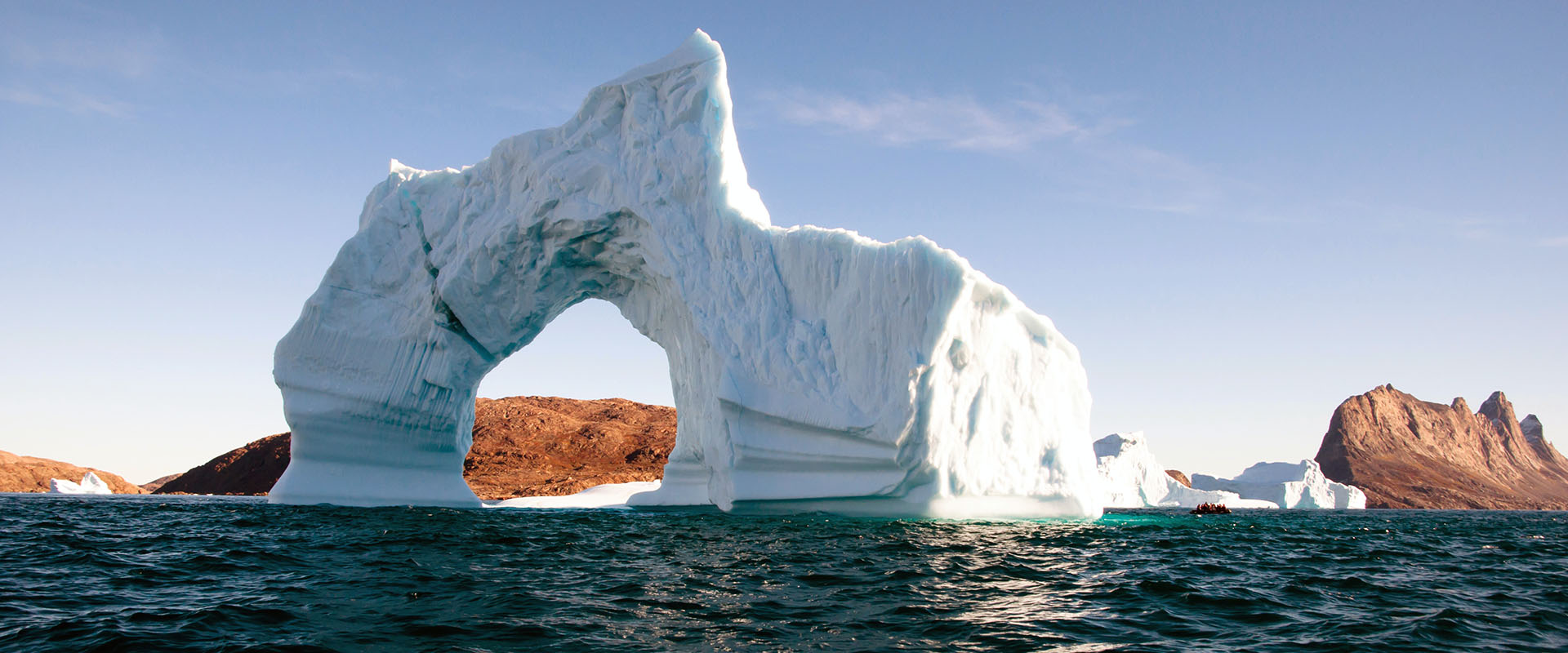The image is a wide, rectangular outdoor photograph taken during a bright, sunny day with a clear blue sky and a few wispy clouds. Dominating the middle of the picture is a massive white iceberg with a significant arch-like hole, resembling a jagged donut or wheel through which the background is visible. The dark, choppy waters beneath it contrast sharply with the iceberg's stark whiteness. Behind this central formation, more white icebergs and barren brown mountains can be seen. On the right side of the image, a small boat with a few people on board provides a sense of scale, underscoring the immensity of the scene. The landscape appears cold, with the bright sunlight reflecting off the water and the iceberg, creating a dazzling effect.